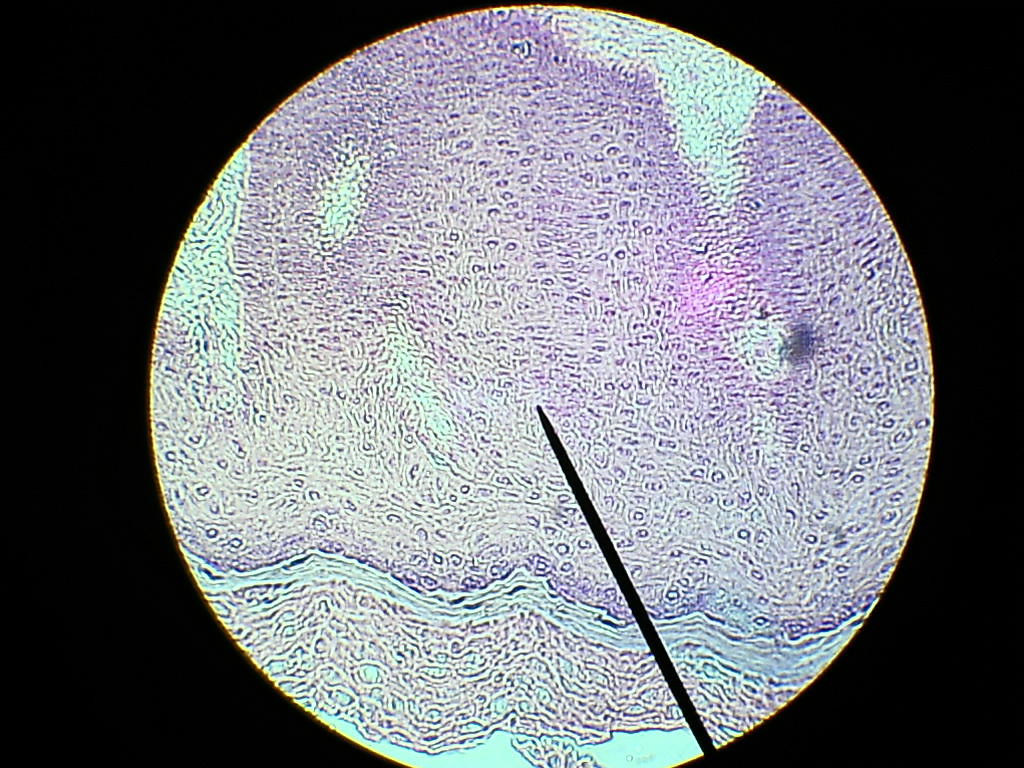This image captures a laparoscopic or microscopic surgical procedure set against a completely black background, creating a stark contrast. Dominating the center is a purplish, circular area of what appears to be biological tissue, exhibiting various recesses and fluid-filled cells. Interspersed throughout the tissue are whitish patches that could indicate different textures or components. The circular tissue surface also features an irregular bump and an intricate design that further enhances its textured appearance. A prominent black line extends through this circular area, likely depicting a vein or boundary between different tissue sections. From the lower right-hand corner of the circular image, a dark, pointed rod, resembling a needle, can be seen being injected into the tissue, indicating an active surgical intervention.